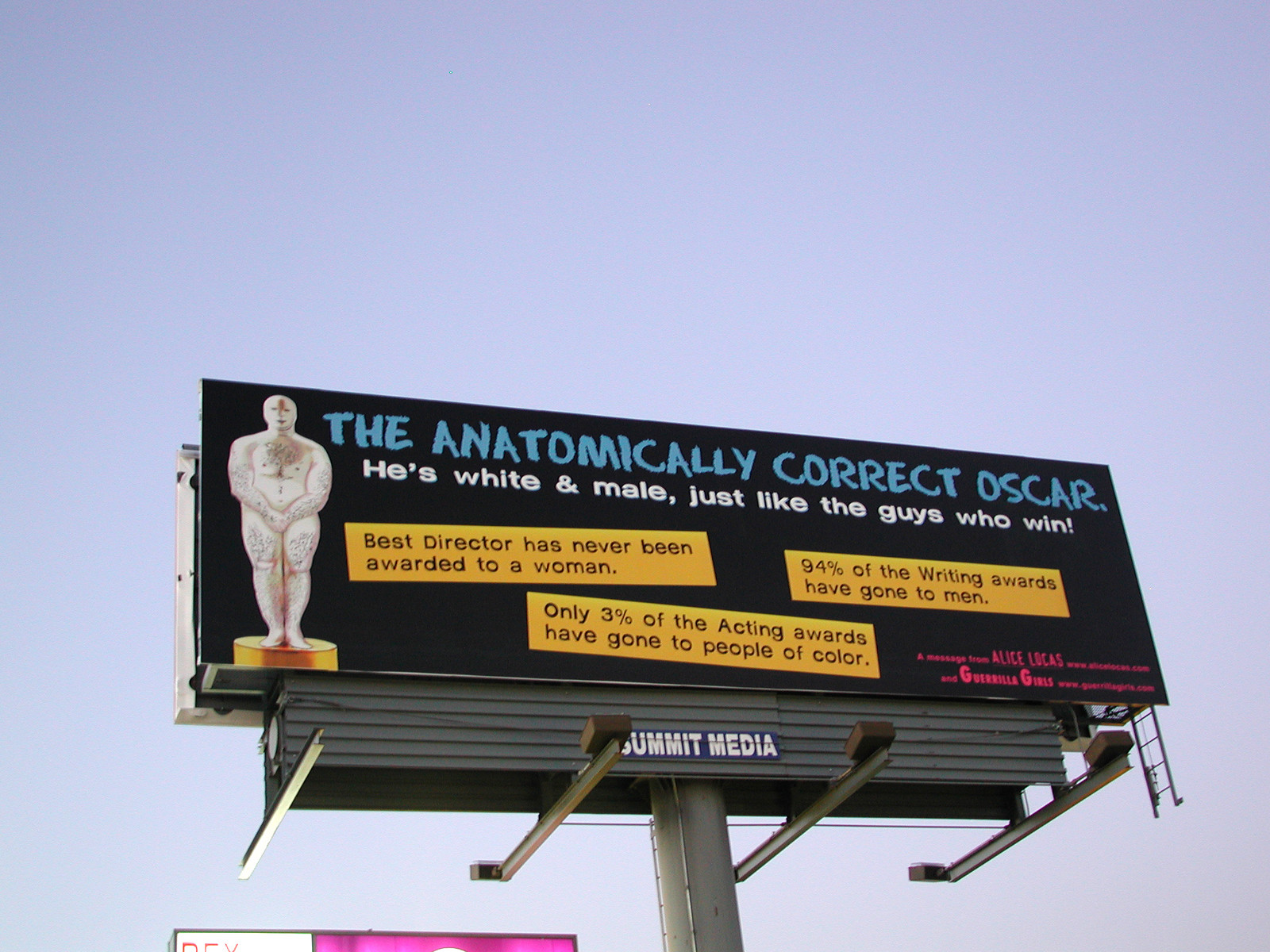In this detailed photograph taken outdoors against an overcast, purplish-blue sky, the main focus is a large billboard featuring a provocative message. The billboard, held up by a weathered, light gray cylindrical pole with additional metal rods for support, stands prominently in the image. The billboard itself has a black background with bold cyan text reading "THE ANATOMICALLY CORRECT OSCAR". Below it, white text proclaims, "HE'S WHITE AND MALE, JUST LIKE THE GUYS WHO WIN." Further down, three long rectangular yellow boxes with black text state: "BEST DIRECTOR HAS NEVER BEEN AWARDED TO A WOMAN," "ONLY 3% OF ACTING AWARDS HAVE GONE TO PEOPLE OF COLOR," and "94% OF WRITING AWARDS HAVE GONE TO MEN."

To the left of the text is a striking statue resembling the Oscar award, but unlike the traditional gold figure, this statue is depicted as a naked white man with dark hair on his arms, chest, and legs, covering his genital area with crossed hands. The statue stands on a gold platform, adding a contrasting splash of color to the dark backdrop.

Above the billboard are small brown boxes attached to metal rods, presumably for nighttime illumination. Behind the main billboard, additional structural elements, including a small gray rectangle, add to the sign's support. Despite some partially cut-off text, the billboard includes a message at the bottom from Alice Lucas, with her name and website URL. The scene is complemented by an additional, mostly obscured billboard in the bottom left, featuring pink text on a white background framed by a black border.